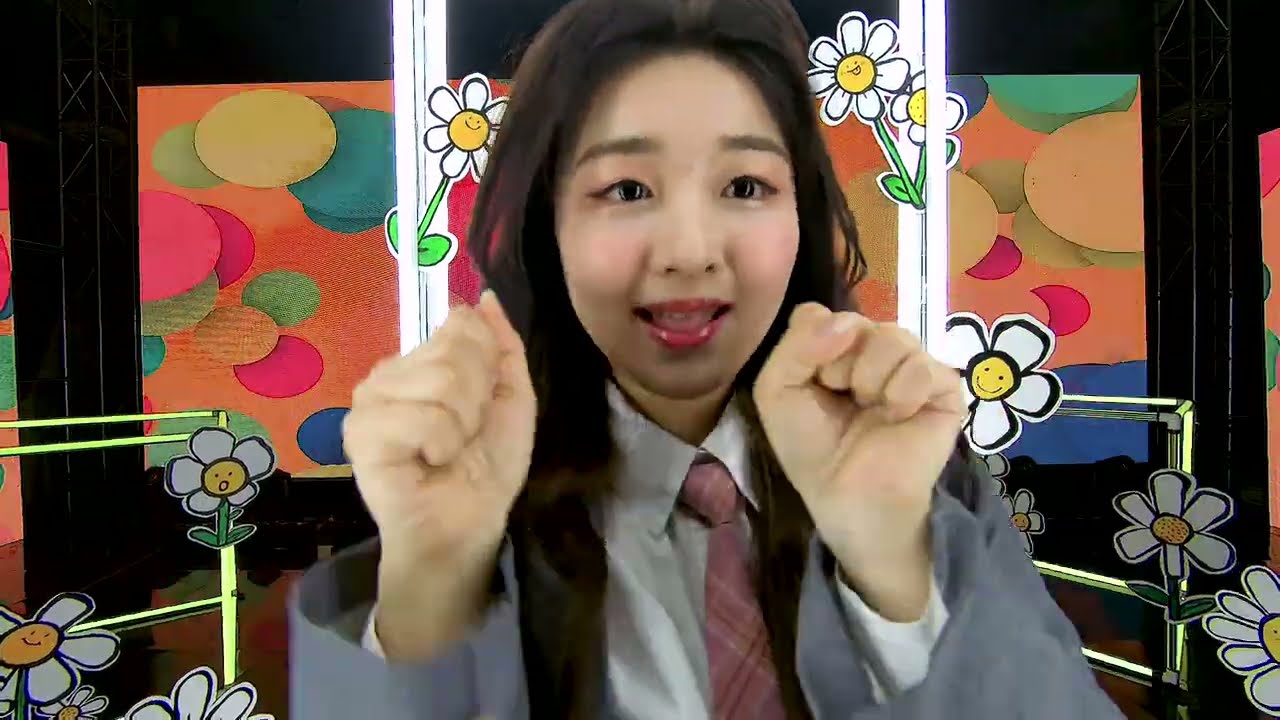This photograph captures an energetic young Asian woman with long, flowing dark brown hair cascading past her chest. Her dark eyes and pink lipstick compliment her pale skin, creating a striking appearance. She exudes a sense of excitement and cheerfulness, as demonstrated by her raised, clenched fists, though she is clearly not angry. She is dressed in a white-collared shirt complemented by a pink, maroon, or reddish tie with subtle orange or darker striped patterns. This ensemble is paired with a gray blazer and layered with a black jacket, giving her a sophisticated, schoolgirl-like look.

In the background, whimsical elements add a playful touch: a series of cartoonish white-petaled, yellow-centered daisies with smiling faces are scattered behind her. These drawn flowers are part of an intricate backdrop that also includes colorful circles and balloons in hues of yellow, green, pink, blue, and purple, all on a predominantly orange background. Additionally, gold metal railings flank her on both sides, and some vertical white bars with more of those cheerful daisies seem to emerge just above her shoulders. This detailed image, possibly a screenshot from a video as suggested by its pixelated quality, captures a vivid, joyful moment brimming with vibrant details and cheerful elements.